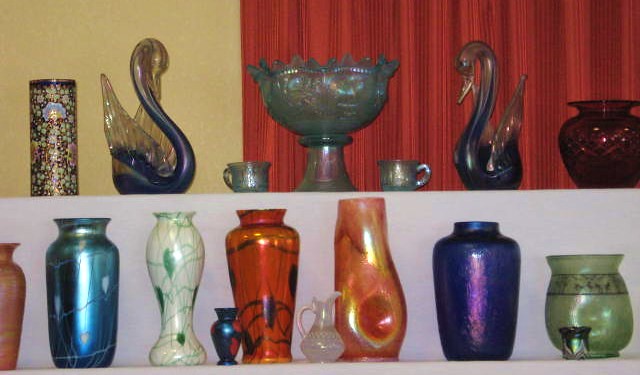This image, likely an older photograph due to its grainy quality, features a two-tiered display shelf adorned with a collection of vintage glass and pottery artifacts from the 1930s to 1950s. The top shelf showcases two striking glass swans, crafted from blown purple glass with iridescent clear glass accents, indicative of the 1940s era. Among these elegant swans is an iridescent turquoise crystal bowl. Flanking them are various stained glass items including a multicolored cup and a large goblet. The backdrop is highlighted by luxurious red curtains, adding depth and contrast to the display.

The bottom shelf is lined with an array of vibrant vases, predominantly featuring the iridescent shimmer that was popular in mid-20th century glassware. Notable pieces include a red vase with black accents and an orange vase adorned with black illustrations. Additional items are a lightning blue vase, a green and white striped vase, a dark lightning blue vase, and vases in hues of pink, blue, and purple. There are also earthy brown clay pottery pieces and a white crackled vase. Enhancing the eclectic collection is a unique piece of radioactive glass, known for its glowing green appearance. Each artifact, with its distinct design and color, contributes to a captivating presentation of historical glass art.